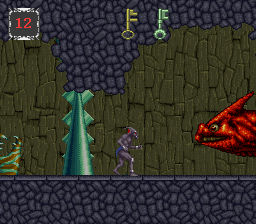This detailed drawing appears to depict a scene from a video game, set against a wall of dark green rocks. The backdrop is intricately textured with jagged green stones, and accented by clusters of purple rocks at both the top and bottom edges. At the center bottom of the image stands a purple character, resembling a man wearing a mask, exuding an aura of mystique. To his left, a serpentine figure ascends, seemingly the tail of a green dragon adorned with menacing spikes. On the far right side of the illustration, the head of a red fish is visible, characterized by a singular horn perched atop its head and a striking red eye. The top left corner of the image features the number 12 in bold red digits, encased within a clean white square. Crowning the piece, two keys, one yellow and one green, are prominently positioned at the top center, suggesting they might be crucial elements or objectives within the game's narrative.